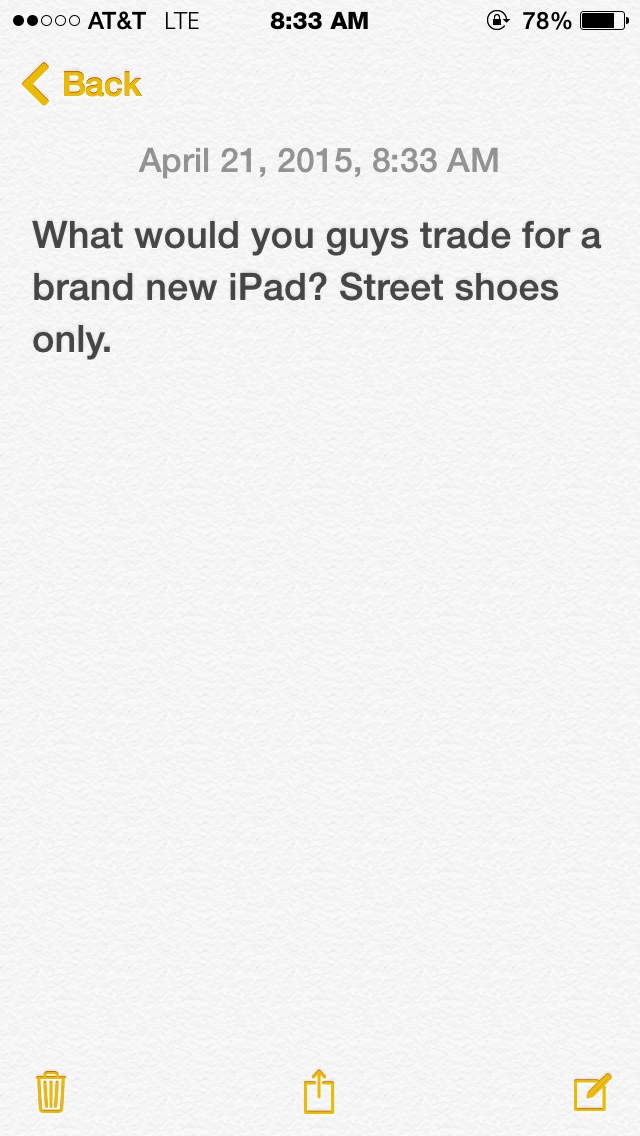The image is a detailed screenshot from an iPad displaying various interface elements. In the upper left corner, "AT&T LTE" is displayed next to five dots indicating signal strength, with two dots filled in black. The top center shows the time "8:33 AM," while the upper right corner displays a battery icon at 78% capacity. On the screen itself, a prominent yellow "Back" button with a left-pointing arrow is visible. Directly beneath this button, the grey text reads "April 21, 2015, 8:33 AM." Below the date and time, a black text message asks, "What would you guys trade for a brand new iPad? Street shoes only." The background of the screen has an appearance reminiscent of a freshly varnished whitewashed wall or old paper. At the screen's bottom, there are three icons: a trash can symbol on the bottom left, a square with an outward arrow in the middle, and a square with a pen symbol on the bottom right.